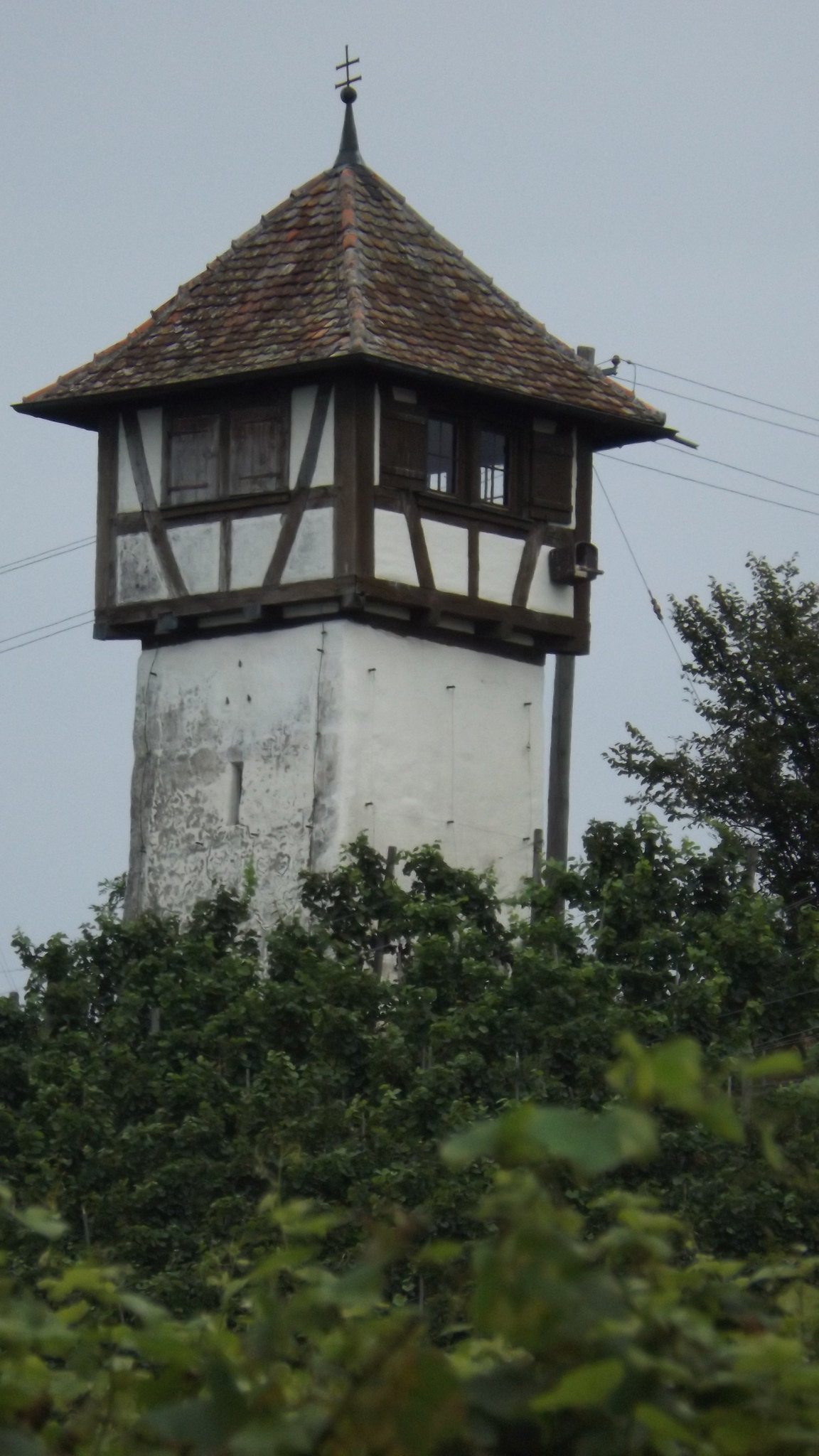This captivating outdoor daytime photograph, presented in a tall, rectangular portrait orientation, captures the striking image of a white rectangular-shaped tower rising majestically above a forested area. At the bottom third of the image, the lush tops of green trees create a vibrant foreground, with lighter-colored leaves in the forefront transitioning to darker hues higher up. The tower itself is an architectural marvel of Tudor-style design, characterized by its white stucco façade with dark brown wood trim adorning the upper half.

The tower's pinnacle features a steep, slanted roof covered in brown tiles, culminating in a small spire topped with a ball and cross. Windows punctuate the white tower just below the roof, set within brown-painted trim, adding to its medieval and watchtower-like design. A network of power lines stretches across the background, subtly visible behind the tower. The sky above is a gradient of gray, hinting at overcast conditions, which gradually transitions to a light blue as it nears the tree line, completing the serene yet imposing scene. Such meticulous details, alongside the representational realism of the photograph, render this image a stunning portrayal of the tower set against its natural and human-made surroundings.